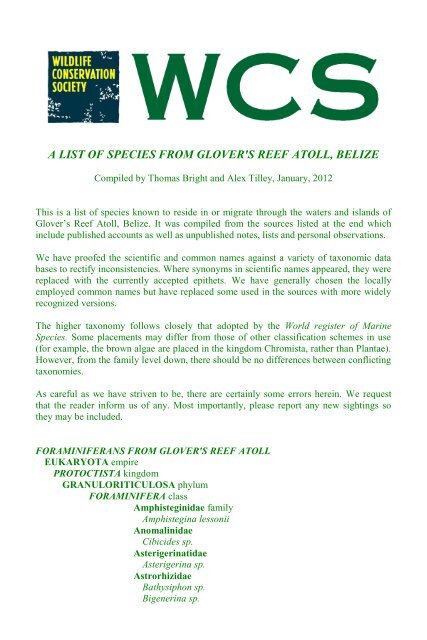This flyer, created by the Wildlife Conservation Society, prominently features their square logo in the top left corner, with yellow lettering on a navy blue background and intricate white details. Next to the logo, the bold green letters "WCS" mark the top of the flyer, which is titled "A List of Species from Glover's Reef Atoll, Belize." Compiled by Thomas Bright and Alex Tilley in January 2012, the flyer contains a detailed description spanning four paragraphs about the reef and the various species that inhabit it, including information on endangered species that need protection. The document concludes with a concise, bullet-point style summary, discussing geographical locations and other critical details about Glover's Reef Atoll.